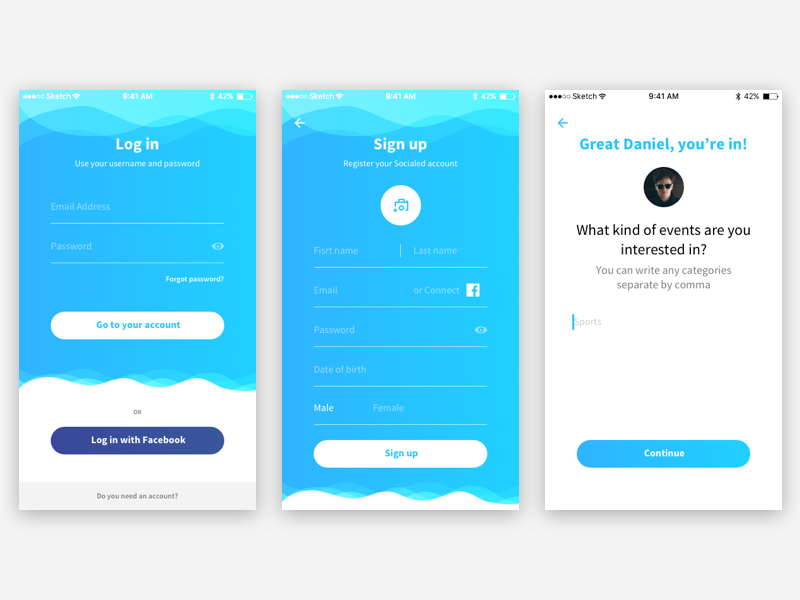The image features three distinct screens, each with a different interface set against a gray background. 

1. **Left Screen**: Dominated by a turquoise, wavy design, this screen serves as a login page. At the top, it prompts users to "Login" and provides fields to enter their email address and password. Below these fields, there is an option that says "Forgot password?". The bottom part of the screen hosts a white button labeled "Go to your account" and a blue button for "Login with Facebook".

2. **Middle Screen**: Similar in design to the left screen, this one focuses on the registration process. The title at the top reads "Sign Up" and below it, "Register your account" (though part of the text is obscured). Users are prompted to input their first name, last name, email, and create a password. The "Sign Up" button at the bottom is white.

3. **Right Screen**: This screen congratulates the user with the message "Great, Daniel! You're in." It displays a profile picture of a person wearing sunglasses. Below this image, there is a prompt asking, "What kind of events are you interested in?" Users are instructed to list categories separated by commas. At the bottom, there is a blue "Continue" button.

This detailed description captures the essence and layout of each screen, highlighting the user interface elements and their functionalities.